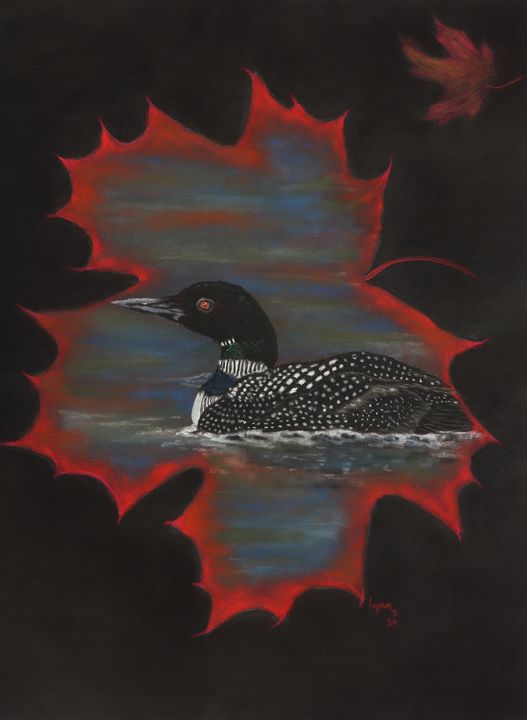The image depicts a brightly colored scene centered on a black background featuring the vivid outline of a red maple leaf. Within this leaf outline, a strikingly detailed illustration shows a black-and-white duck with a distinct black head, highlighted by orange eyes and a pointed black beak. The duck's body bears black-and-white spotted patterns, with additional subtle hues of green, blue, and white around its neck, creating an exotic appearance. It is depicted in water with swirling colors of red, orange, blue, green, and white around it, adding to the vibrant detail. The scene suggests the appearance of a mallard with a grey beak. There is also a much smaller, entirely colored maple leaf located in the top right corner, contrasting the larger outlined leaf. At the bottom right of the image, there is a small red signature reading 'Lin' with some additional, unreadable marks appearing to include the year '20'.